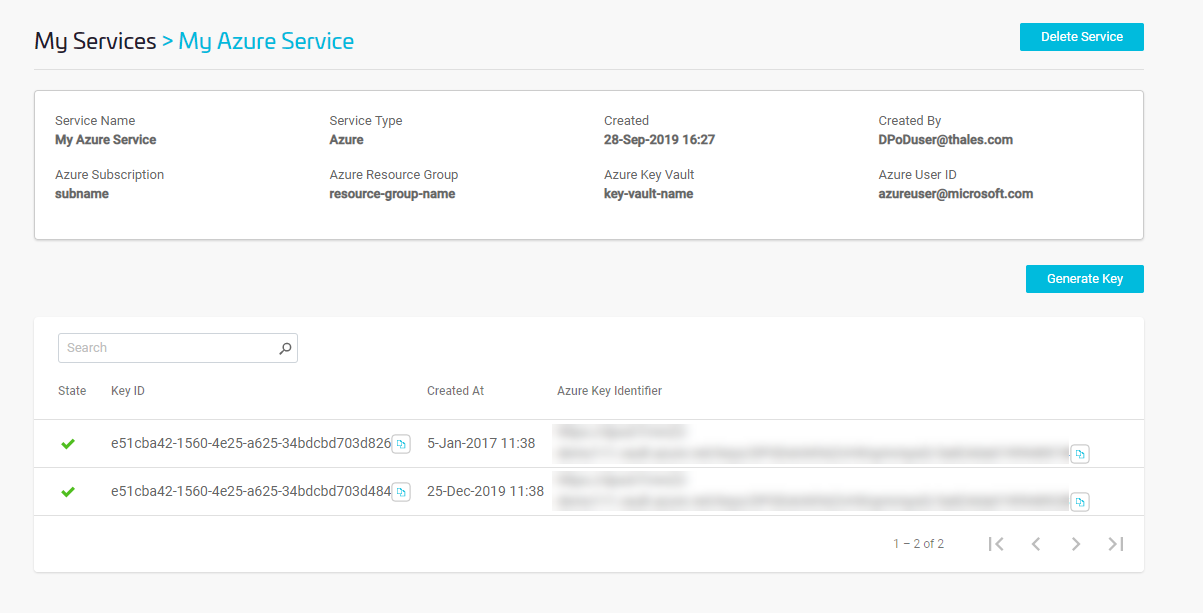In this image, the top section is adorned with a light blue background featuring the title "My Services." Beneath it, a blue arrow pointing to the right leads to the label "My Azure Service." Situated in the right corner, a blue "Delete Service" button is prominently displayed.

Central to the image is a white box with a blue outline containing detailed service information. It lists:
- **Service Name**: My Azure Service
- **Service Type**: Azure
- **Created**: 28th September, 2019, 16:27
- **Created By**: depoduser at fails.com
- **Azure Subscription**: Subname
- **Azure Resource Group**: Resource Group Name
- **Azure Key Vault**: Key Vault Name
- **Azure User**: azureuseratmicrosoft.com with an associated ID

Below the white box, there is a blue box containing a blue "Generate Key" button.

Further down, a search box with multiple fields is visible, including:
- **State**
- **Key ID**
- **Created At**
- **Azure Key Identity**

Two lines with green check marks display additional details:
1. **ID**: [Hidden], **Date**: 5th January, 2017, at 11:38
2. **ID**: [Hidden], **Date**: 25th December, 2019, at 11:38

The key identifiers are blanked out for privacy reasons. At the bottom of the image, a pagination section shows "2 of 2" along with navigation arrows flanked by separator lines enabling users to switch between pages.